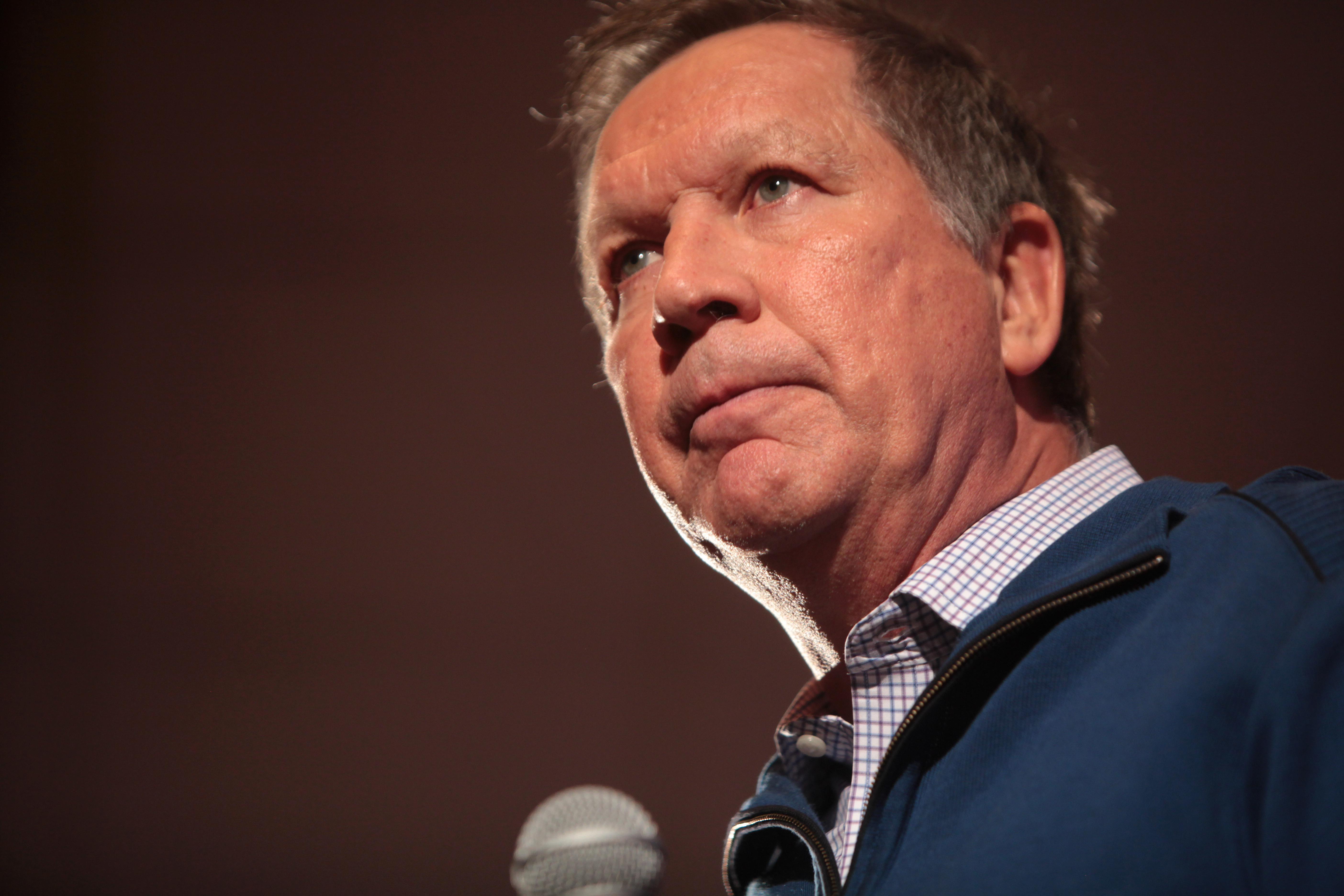In this photograph, an older Caucasian gentleman stands against a brown backdrop, likely speaking at an event or press conference. The image captures him from a close, upward angle, emphasizing his serious expression as he looks slightly off-camera to the left, evidently concentrating on something being said to him. The man holds a microphone, which is barely visible at the bottom left of the frame. He has short, tussled gray and white hair, with very subtle or barely visible eyebrows that are likely light in color. His medium blue eyes are hooded but alert, adding to his intense demeanor. He is dressed in a cadet blue jogger-type jacket over a button-down shirt that primarily white with a grid of blue lines forming squares. There is a notable contrast in lighting, with a heavier illumination on the lower left side of his face, softening as it goes upward.